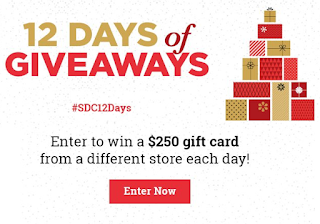A festive pop-up advertisement appears on the screen, titled "12 DAYS OF GIVEAWAYS" in bold, all-caps font, with "12" numerically represented and "DAYS" in antique gold. The word "of" stands out in a cursive, berry-red italicized font. Below this, the word "GIVEAWAYS" is displayed in muted red, also in all caps. Toward the bottom, the hashtag #SDC12DAYS is prominently featured next to an image of a neatly stacked collection of presents, wrapped in various shades of antique gold and red. Beneath this, a call-to-action text invites viewers to "Enter to win a $250 GIFT CARD from a different store each day." The overall design clearly evokes a holiday theme, encouraging immediate participation in the daily gift card giveaway contest.